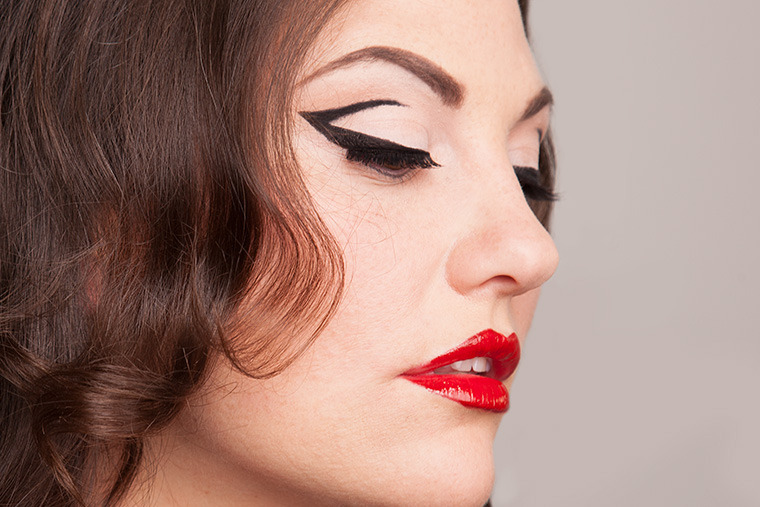This close-up photograph captures the striking visage of a fair-skinned woman, prominently displaying the features from her chin to her forehead. Her head is slightly turned to the right, revealing a cascade of brown hair falling alongside her left cheek. The focal point of her face is accentuated by bold, red lipstick that highlights her partially open mouth, showcasing her top teeth. A dramatic touch is brought to her eyes, which are adorned with thick, black fake eyelashes and meticulously applied eyeliner that curves like a bracket, emphasizing the allure of her half-closed eyes. The backdrop on the right side of the image is a simple gray, providing a neutral canvas that draws attention to the intricate details of her facial features. The overall ambiance creates an impression of contemplative elegance.